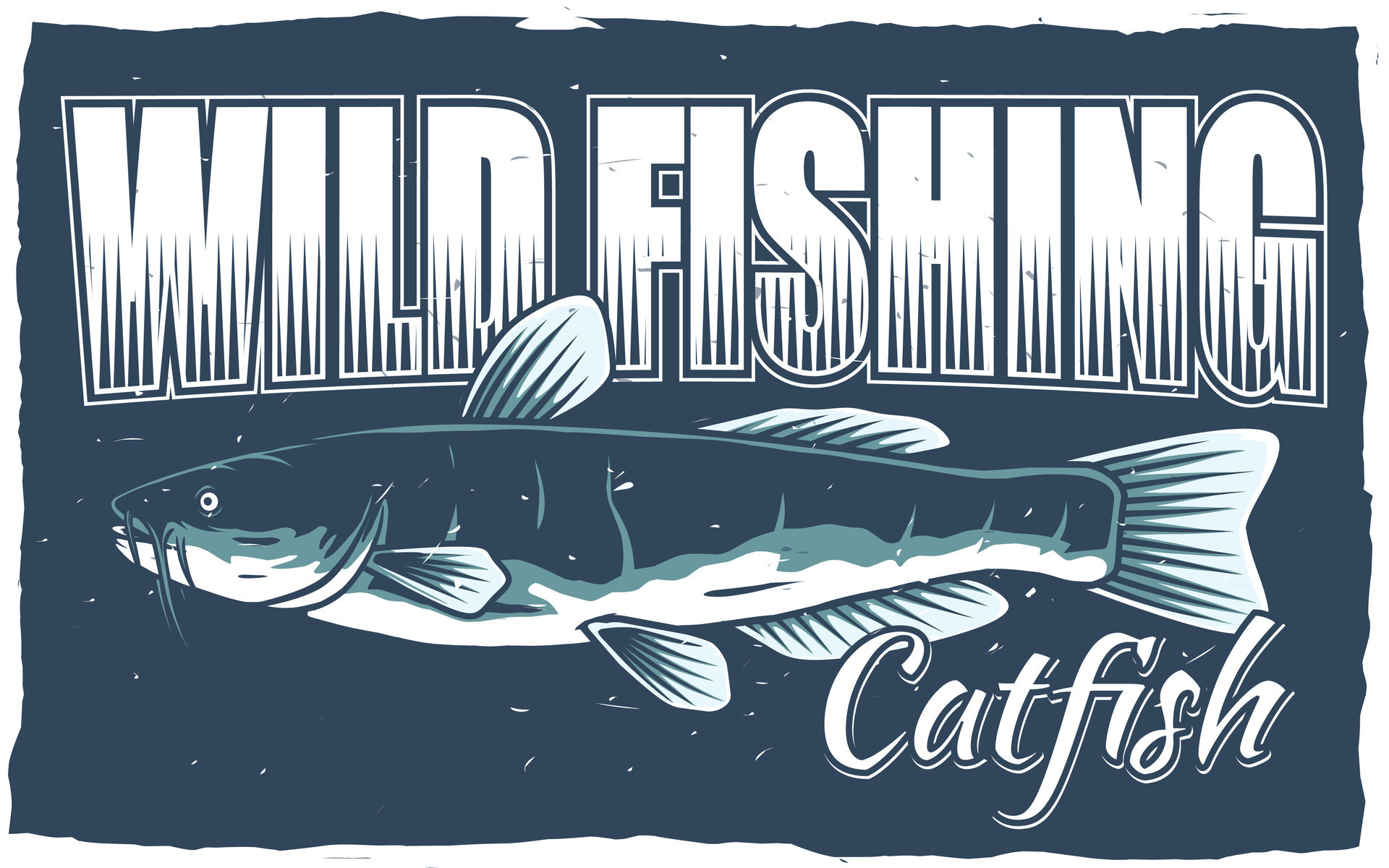This is an illustration with a rugged-edged background, not perfectly rectangular, in a dark bluish-gray color. Bold, large white letters with a dark blue outline at the top spell "Wild Fishing," with stylized stripes rising up the bottom half of each letter in the background's hue. Below this text is a prominent image of a fish, resembling a trout or catfish, depicted in the same dark blue-gray as the background but distinguished with a lighter outline. The fish has six fins including the back fin, lighter fins and tail outlined in white, and shading inside matching the blue-gray theme. It is shown facing left with long whiskers extending from the front. At the bottom right of the illustration, "catfish" is written in white letters. The elements suggest it may serve as a logo or advertisement for a company offering wild fishing, specifically highlighting catfish.